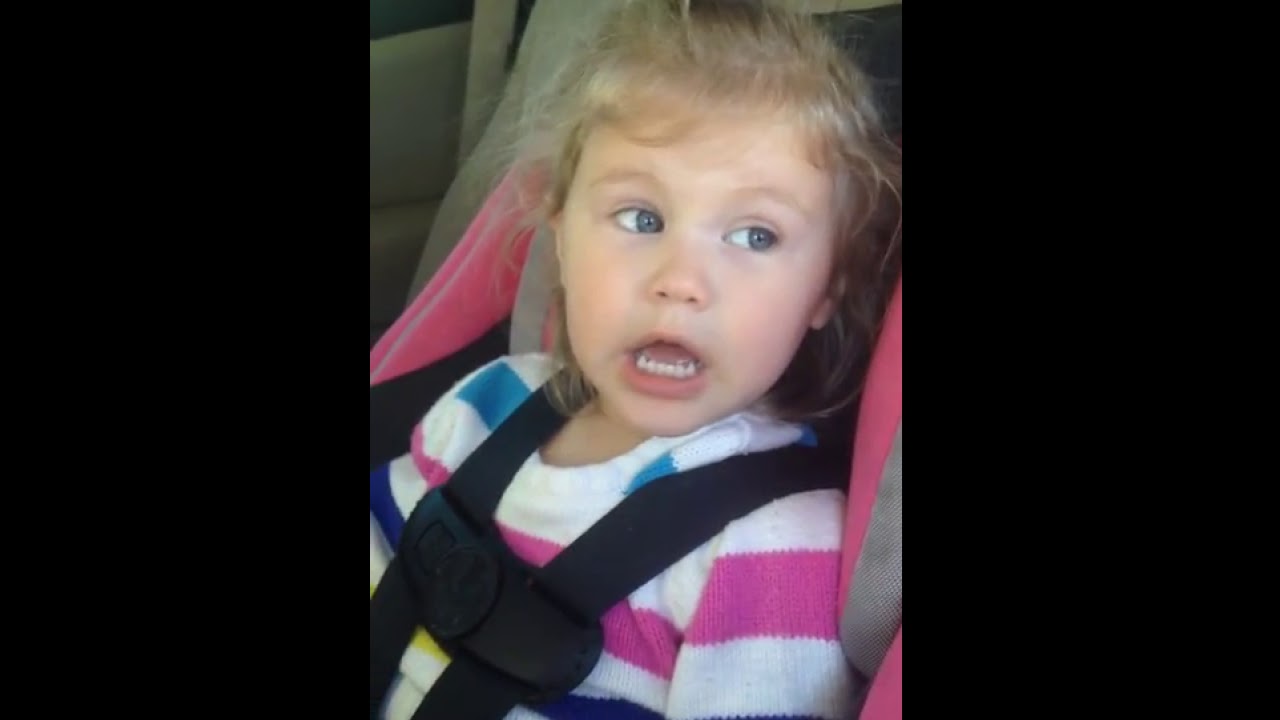In the center of the image, a toddler with blonde hair, blue eyes, and bangs is seated comfortably in a pink and gray car seat, secured by black straps. She appears to be a little over two years old, judging by her full set of visible lower baby teeth. The child is wearing a white shirt with bright blue and pink stripes. Her eyes are wide open as she looks off to her left side, her mouth open as if she is speaking or perhaps singing. The background on either side of the photograph is black, emphasizing the child's focused expression and lively demeanor as she interacts with someone, possibly outside the car window or within the vehicle.